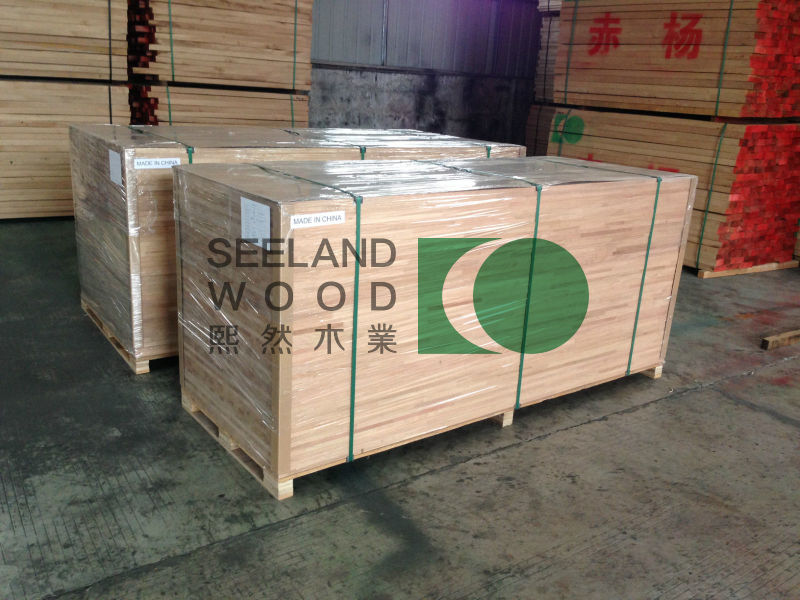The image depicts a warehouse setting that appears to be either in China or a location that imports Chinese goods. The focal point is on two large wooden pallets wrapped in plastic, labeled with "Sealand Wood" in black capital letters, accompanied by Chinese characters beneath. The centerpiece of the logo features a green circle alongside a green rectangle with a semi-circle cut out, which appears stamped onto the image. The pallets are situated on a worn concrete floor, consisting of large gray slabs that show signs of discoloration. Stacked wooden planks are visible behind the main pallets, divided into sections with red edges and red stamped Chinese characters. Additional stacks of tan wood, divided into segments by orange markings and another green logo, are visible in the upper left section of the image, highlighting the industrial environment.